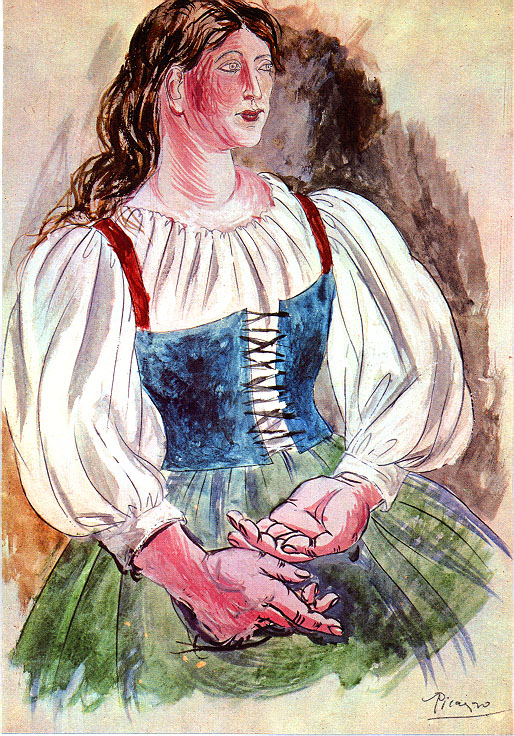The image depicts a Picasso painting or drawing in the lower right-hand corner, characterized by less abstraction than many of his works. The subject of the painting is a woman, possibly a peasant, seated and gazing pensively off to the right. She is adorned in a complex outfit consisting of a green skirt, a blue corset laced with black tie and red stripes, and a voluminous white peasant blouse exposing her neck. The woman’s long, wavy brown hair flows down her back and is complemented by a comb behind her ear, with her rounded face featuring red lips and oval eyes.

Her unusually large hands are prominently stylized – the left hand is extended towards the viewer with an open palm, while the right hand is more relaxed, showcasing the back of the hand and visible veins. The background transitions from a darker brown behind the woman to a softer beige further back, creating depth and focusing attention on her contemplative expression and distinctive attire. Testament to Picasso's signature, the painting captures both an intimate and exaggerated portrayal, almost resembling a caricature in its emphasis on certain features like the hands and the warm tones of the woman’s face.